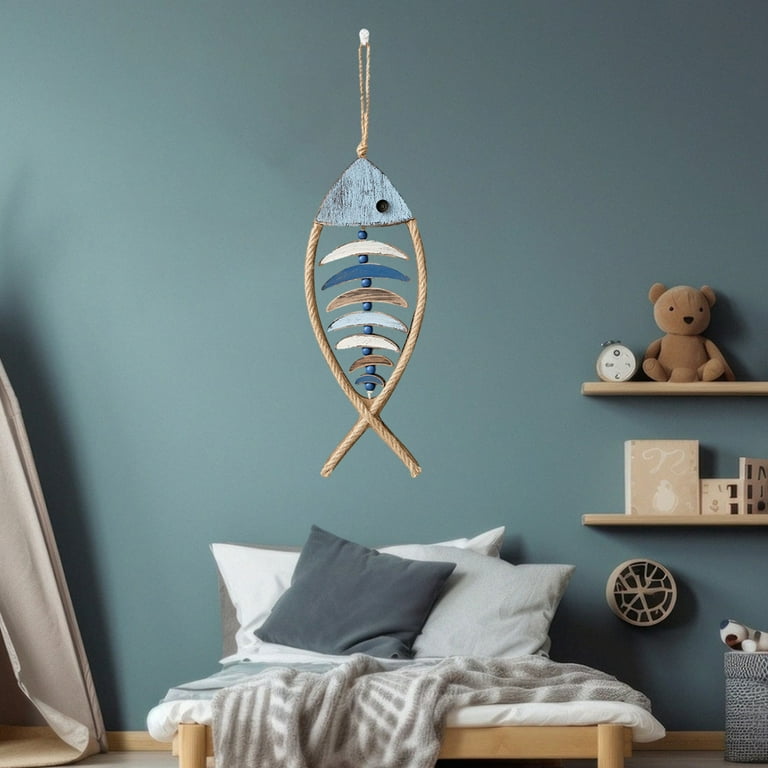The bedroom in the photo features an unmade bed with a tangled comforter, flanked by a blue pillow and several white pillows, all set against a wooden frame. The wooden stand holds a small tent. Above the bed, suspended from the ceiling, is a stylized fish crafted from rope, with its head hooked onto a thumbtack and a black eye. The fish's body is defined by descending ropes, each diminishing in size to represent the ribs, accompanied by different chimes. Beyond the bed, a blue wall with wood trim along the bottom frames the scene, with a white carpet below. On one side, a shelf displays a clock, a teddy bear, and what appears to be a small box or a fake front of a building. Another shelf holds various books. A little circle decorates the area above the bed, accentuated by a gray square featuring an animal.